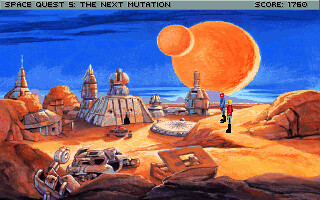This image is a detailed art-style scene from the video game "Space Quest 5: The Next Mutation", reflected in a small pixelated form with an old-style, DOS game feel. At the top of the image, a light gray banner displays the game's title and a score of 1760. The setting is an apocalyptic, desert-like planet with a striking, dark blue sky. Dominating the sky are two large, orange-yellow celestial bodies: a large one with a smaller one overlapping it slightly. The foreground features a variety of futuristic debris, including what might be car junk, a large partially opened box, and possibly robots. Two human figures stand atop a stylized, rocky mound, seemingly interacting with the environment. In the background, futuristic buildings and pyramid shapes create a distinctive, otherworldly landscape, including a structure reminiscent of a sultan's futuristic palace. The overall aesthetic of the image exudes an oil pastel or painted look, enhancing its vintage gaming charm.